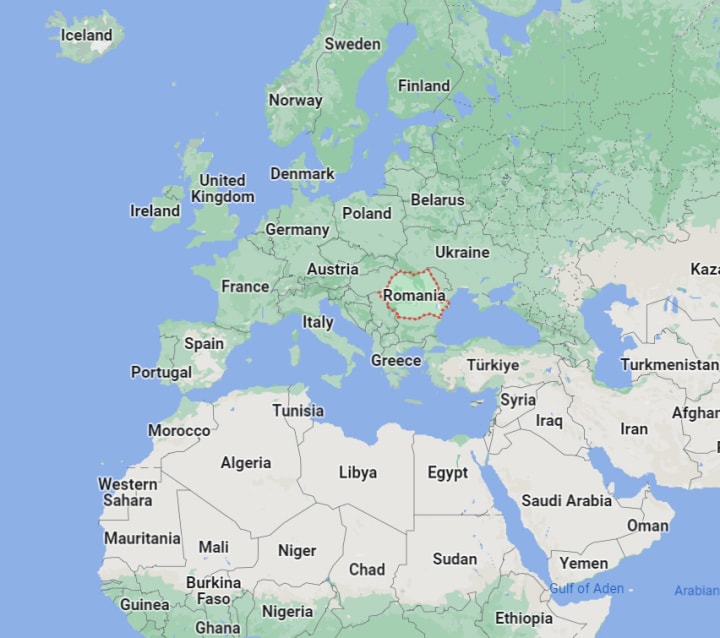The image depicts a geopolitical map covering parts of Europe, Northern Africa, and Western Asia, set against a background of sky blue indicating the ocean. Iceland is positioned at the top left, highlighted in green with its name in black text. Moving towards the center, Romania stands out with its border outlined in a distinctive red dotted line. Surrounding Romania are several neighboring countries, including Ukraine to the right, Poland and Germany to the left, Austria below, and Bavaria above. To the bottom left of Europe lies France and Italy, continuing downwards to Ethiopia, Nigeria, Ghana, and Guinea in Africa. The right side of the map spans over to Iran, Turkmenistan, and a partially visible Afghanistan. The northern part of the map features Sweden, Norway, and Finland, all in their respective colors. Europe and the greener parts of Africa are shaded predominantly in green, contrasting with the whitish, desert-like hues of Northern Africa and the Middle East. Each country is clearly labeled, with Europe and Middle Africa emphasized with a greener palette to indicate lush regions, while the Northern Africa and Middle Eastern regions are depicted in stark, arid tones.